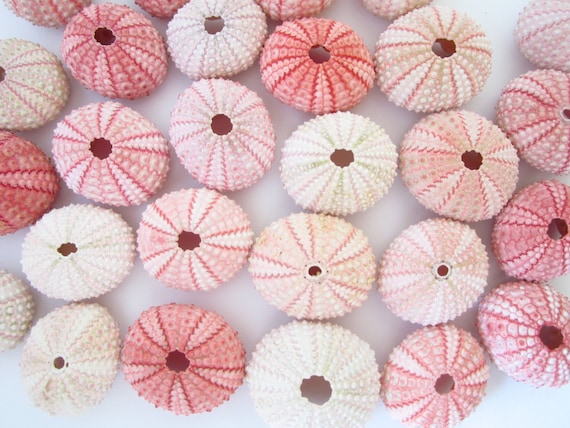This horizontal landscape image features a striking arrangement of empty sea urchin shells set against a stark white background. The shells, occupying the entire frame, exhibit a mesmerizing variety of stripes in shades of light pink, dark pink, white, and coral, resembling the tops of lollipops or pinwheels. These shells, intricately patterned and woven, each have a distinct round shape with a prominent hole in the middle. They are aligned in asymmetrical rows and columns: six in the topmost row, seven in the second, five in both the third and fourth rows, with three shells on the left edge visible only halfway, and four shells along the top edge visible in varying degrees from quarters to almost whole. The detailed pattern and coloration, coupled with the orderly yet uneven juxtaposition, create a visually engaging and detailed display.